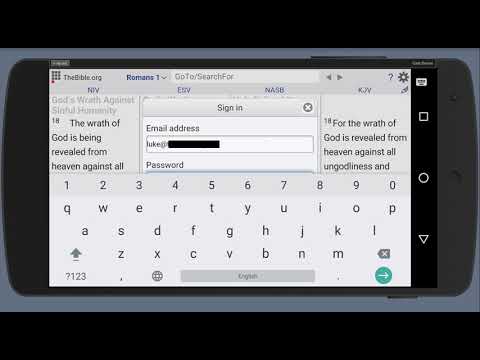The image is a horizontal, left-to-right digital screengrab, likely from a smartphone device. The background is uniformly black, extending in solid, uninterrupted bands at both the top and bottom edges, giving it a flat and one-dimensional appearance. Dominating the center of the image is a slate-gray rectangular section, within which an iPhone display is shown, oriented sideways rather than in the conventional upright position.

On the iPhone screen, multiple browser tabs are visible at the top, including a currently active tab labeled "bible.org, Romans 1." There are options to search different Bible translations such as NIV, ESV, NASV, and KJV. The primary text displayed reads "God's wrath against sinful humanity. The wrath of God is revealed from heaven against all..." which appears to be an excerpt from the scripture.

A prominent pop-up box is overlaid on the screen, prompting the user to sign in. This box contains fields for an email address, "Luke at..." (with the remainder of the email obscured), and for a password, which is not visible. At the upper right corner of this sign-in box, there is an "X" to close it.

To the right side of the screen, there is a vertical sidebar with a partial verse, "18 For the wrath of God is revealed from heaven against all godliness and..." which cuts off abruptly. The upper right-hand corner of the iPhone display also features a question mark icon, likely for help or information, and a settings icon.

At the bottom portion of the screen, the iPhone’s on-screen keyboard is visible, displaying the standard numerical keys (1 through 9 and 0) and a traditional QWERTY keyboard layout beneath it. Running vertically along the right-hand side of the entire image are three standard smartphone navigation icons: a square, a circle, and a triangle, indicating multitasking, home, and back functions respectively.